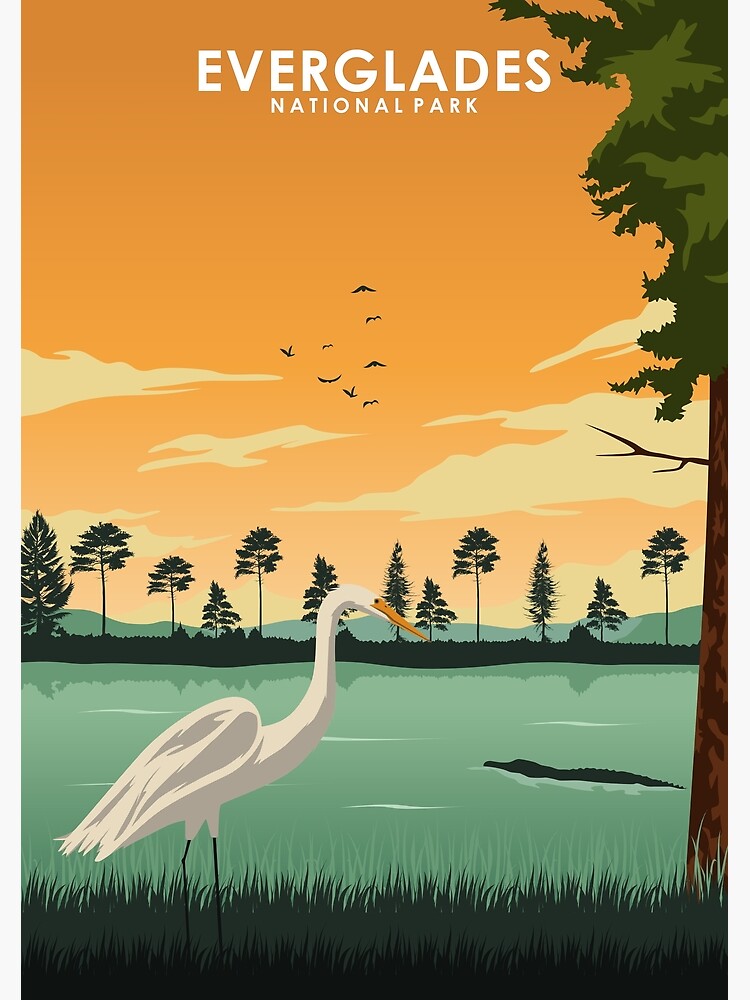This vertical, colorful illustration is a vibrant graphic of Everglades National Park, prominently indicated by white, all-capital letters at the top center. Dominated by oranges, greens, and black hues, the scene captures a sunset over a swampy area with turquoise-blue and green water. In the lower left corner, a tall white bird, possibly an egret or heron, stands upright with long black legs, a gray-dappled chest, and an orange-yellow beak, gazing down at the marshy water beneath it. Nearby, to the right, the head of an alligator can be seen swimming through the water. The scene is framed by tall grass and darkened black pine trees along the horizon. The sky is vibrant orange with yellow-tinged clouds, dotted with tiny black silhouettes of birds in flight. On the far right, a large tree with a brown trunk and lush green foliage stretches from the bottom all the way to the top of the image, completing the serene wildlife setting.